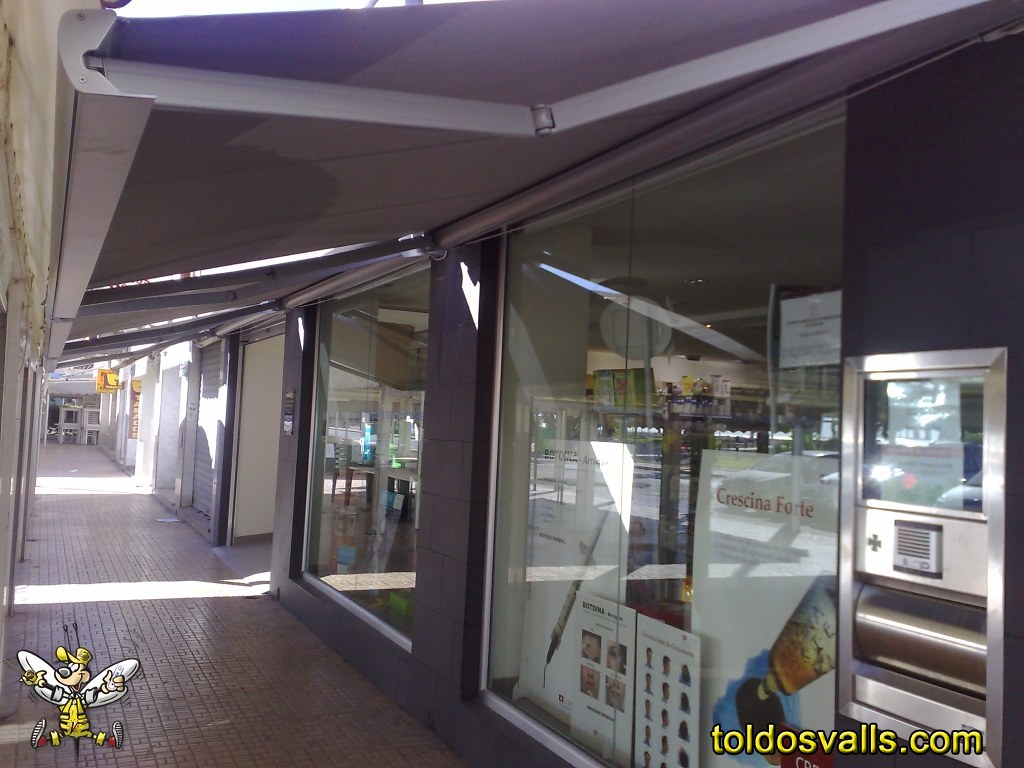The photograph captures the exterior of a strip mall, presented in landscape orientation. The foreground reveals a shaded area, created by a fabric awning that spans across the top of the image, intermittently allowing harsh, bright sunlight to break through in horizontal strips. This lighting effect casts bands of sunlight onto the brick pathway beneath it, which runs down the left side and converges into the distance toward the center left.

The strip mall itself features a series of large glass storefronts on the right, divided by hazy, dusty purple walls. These reflective windows, laden with posters and promotional materials, make it challenging to discern specific products inside, although there seem to be items related to ink or pens displayed. One noticeable poster displays text in a different language, reading "Ciena Forte."

Down this corridor of storefronts, there's an overhead covering providing a shaded environment, protecting from the direct sunlight. Additional details include a possible kiosk or ATM located toward the far right of the image. At the bottom corners, eye-catching elements are present: to the left, a whimsical cartoon character of a yellow bee donning a bee suit, with white wings and spread arms, wearing sneakers and a small hat; to the right, a website URL "toldosvalls.com" is written in yellow letters, hinting at the origin of the image.